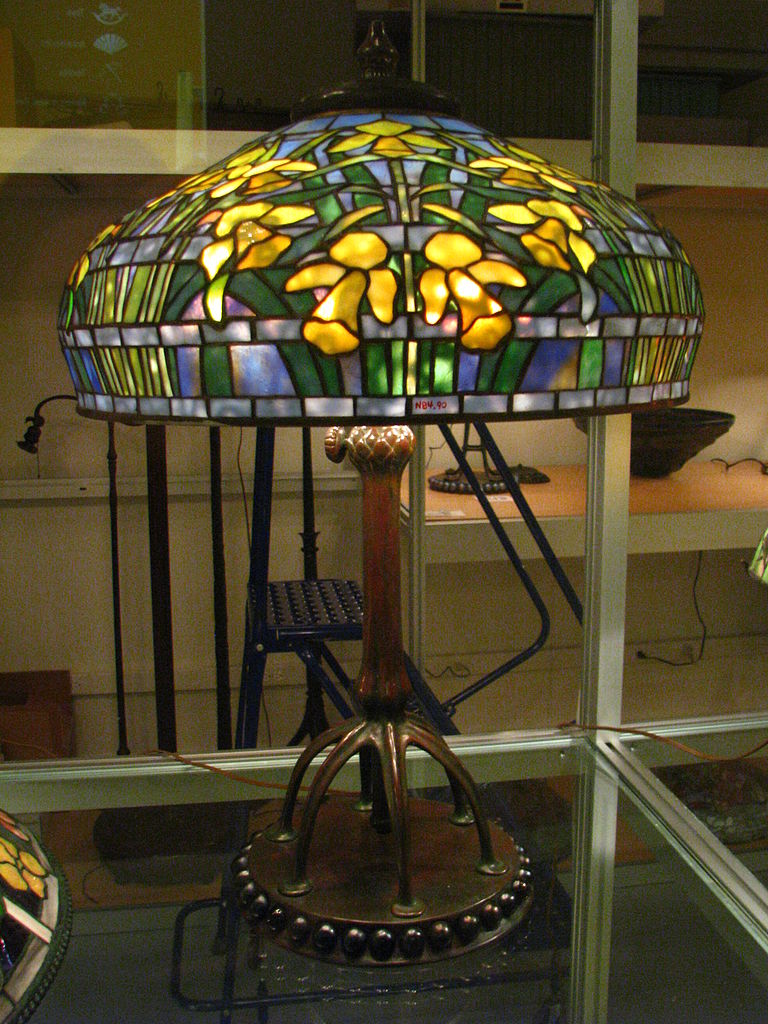This is an image of a Tiffany-style lamp, prominently displayed on a glass shelf or possibly a display case, likely in a shop or museum setting. The lamp's stem is intricately designed to resemble a tree trunk, with roots sprawling onto a circular base adorned with beads of a matching brownish-bronze hue. The shade of the lamp is a masterful display of stained glass artistry, featuring rows of bluish-purplish glass tiles that create a vibrant mosaic. Interwoven within the mosaic are detailed depictions of yellow daffodils, green stems, and leaves, creating a captivating tableau. The art deco-style design showcases a checkered pattern and light opalescent blue squares encircling the lampshade. A reflection visible in the glass hints at the photo being taken through another glass surface. The background includes other mosaic pieces, another lamp with its cover removed, and a small stool, suggesting a setting that could be a repair shop or a display venue.